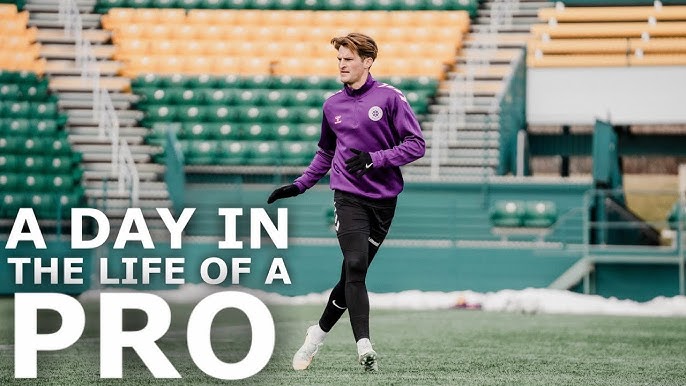A realistic, horizontally oriented photograph captures an outdoor scene at a sports stadium. The stadium, with empty green and yellow seating, is complemented by white staircases and metal railings in the foreground. Snow piles are visible in the background, defining a chilly setting. Dominating the center is a tall, clean-shaven, white male athlete, probably in his 20s or 30s, with short light brown hair. He is wearing a purple tracksuit, black Nike gloves, black athletic pants with white markings, and white cleats. The man is running towards the right side of the image while looking to the left, seemingly mid-jog. White text in the lower-left corner reads, “A day in the life of a pro.”